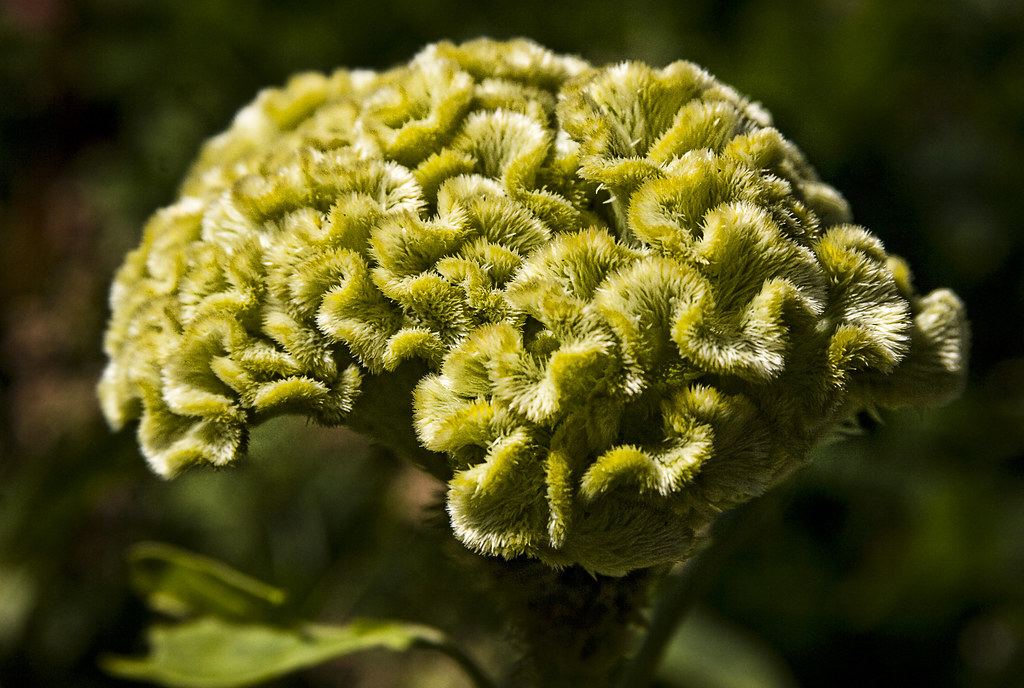This image is a well-lit, outdoor, close-up color photograph of a coxcomb flower, which intriguingly resembles a brain or brain coral. The flower exhibits a mesmerizing pale green hue with goldish highlights and has a bristly, velvety texture. The coxcomb's intricate, winding structure creates dark, shadowy areas that contrast beautifully against the lighter portions. Set against a blurred dark background where faint leaves and stems can be seen at the bottom left, the overall focus remains strictly on the flower, emphasizing its extensive and unique design. The light source, likely from above, casts a gentle illumination that enhances the flower's details, making it the central and sole subject of this captivating image.